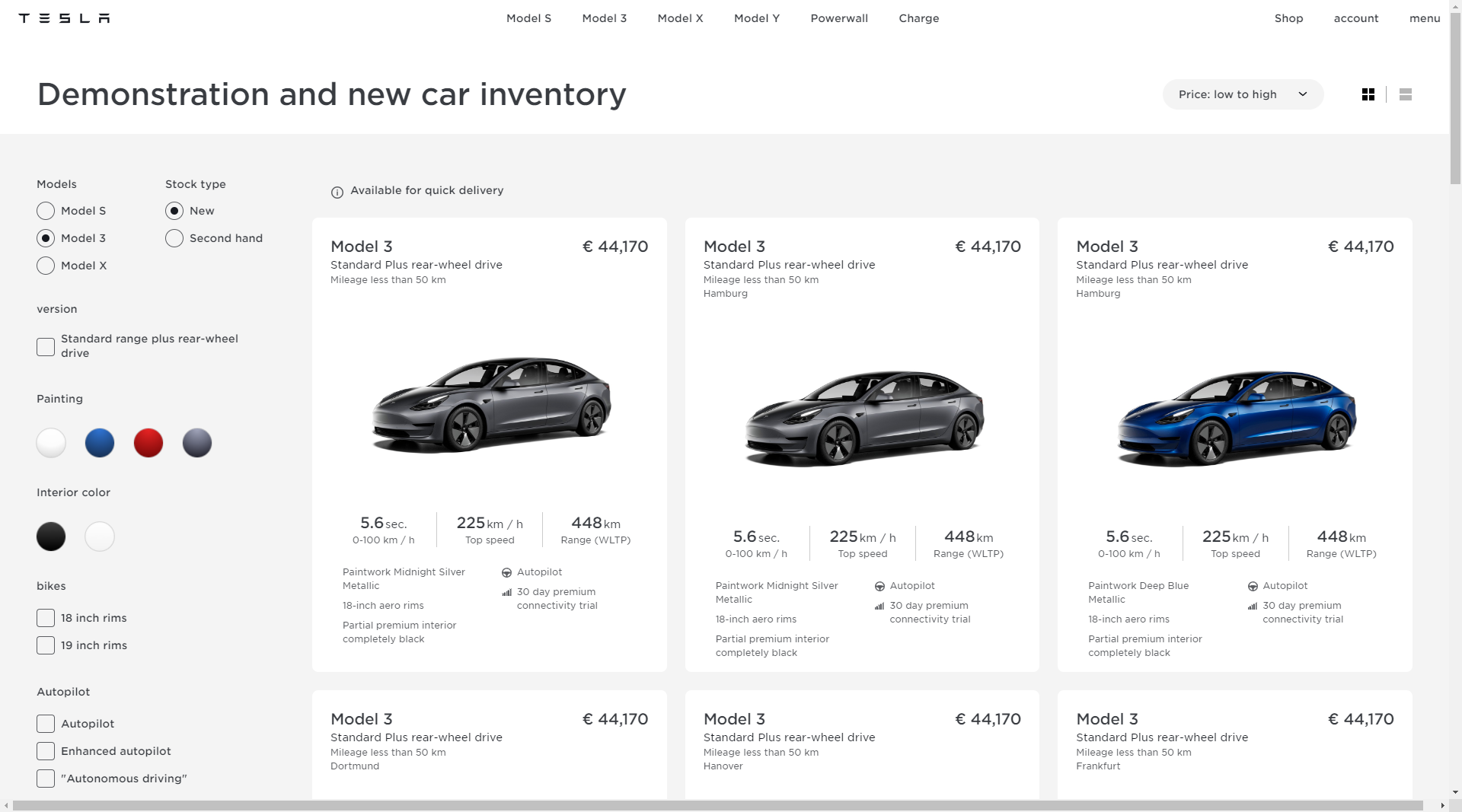The image appears to be a screenshot from a Tesla dealership website. The header prominently features the Tesla logo with navigation tabs for Model S, Model 3, Model X, Model Y, Powerwall, and Charging. Beneath this, there are links for Demonstration and New Car Inventory. The main section showcases three Tesla Model 3 vehicles, two in gray and one in royal blue, each priced at $44,170. Key performance metrics for these vehicles are highlighted: 5.6 seconds acceleration, 225 km/h top speed, and a range of 448 km. 

To the left, a sidebar allows users to customize their vehicle choices by selecting the model and opting for new or secondhand cars. Color options include white, royal blue, red, and gray, with interior choices of white or black. Further customization options include selecting rim sizes and features such as basic Autopilot, Enhanced Autopilot, and Full Autonomous Driving.